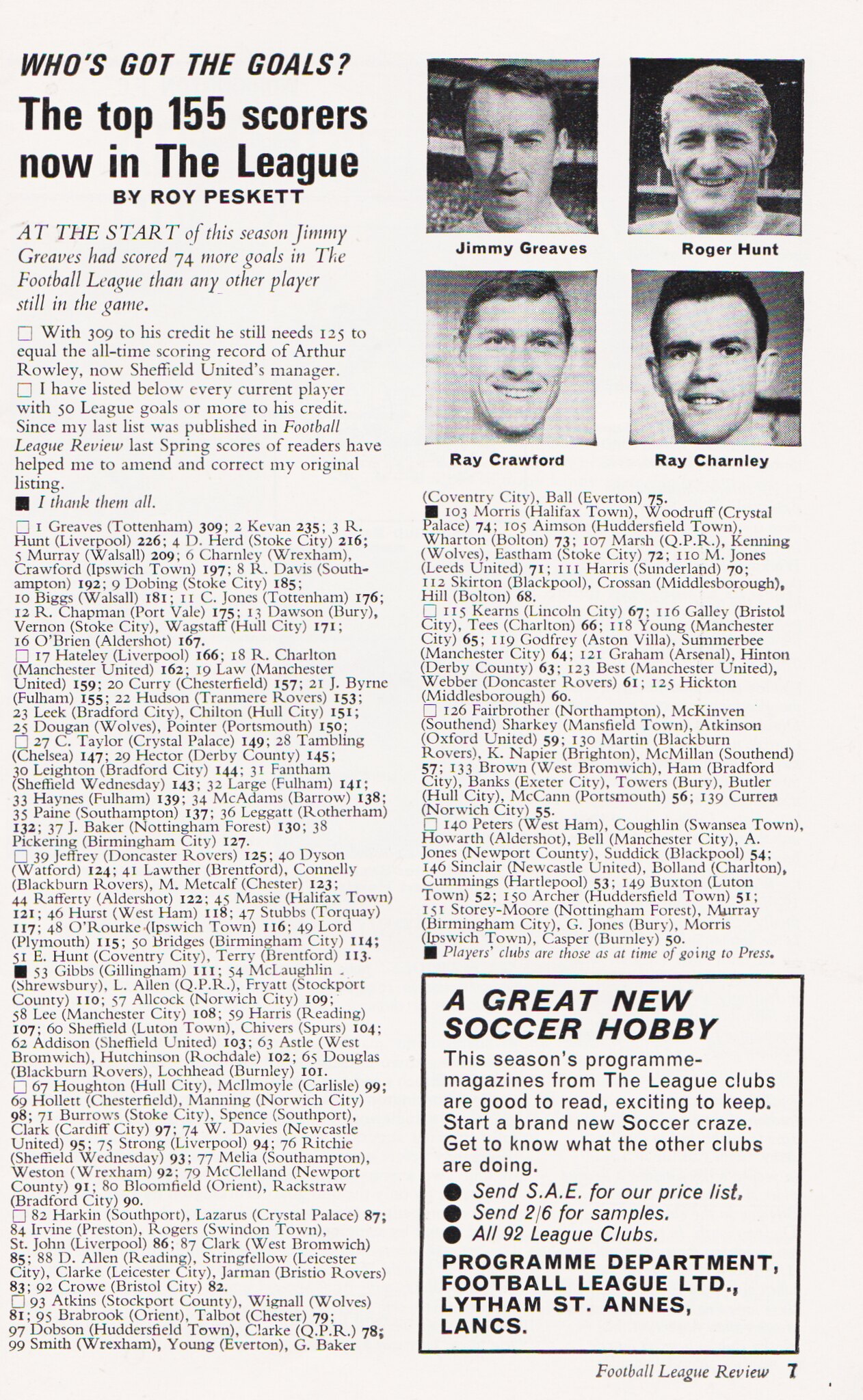This is a meticulously detailed page likely extracted from an older edition of the Football League Review magazine, dated several decades ago. At the top left, a bold heading asks, "Who's Got the Goals?" followed by the main headline, "The Top 155 Scorers Now in the League by Roy Peskett." This article includes an extensive list, ranking the top 155 goal scorers in the English league. Supporting the text are four black-and-white photographs of notable players: Jimmy Greaves at the top left, Roger Hunt to his right, Ray Crawford below Greaves, and Ray Charnley next to Crawford. All four players, clean-shaven and smiling, represent prominent footballers of that era. The detailed list of players and their accomplishments extends down the left column and continues on the right side of the page. Additionally, a box at the bottom right corner promotes "a great new soccer hobby," encouraging readers to collect season program magazines from league clubs. The advertisement includes details on acquiring a price list from the Football League Limited, based in Lytham St. Annes, Lancashire. The footer reveals this as page seven of the Football League Review, published in the United Kingdom.